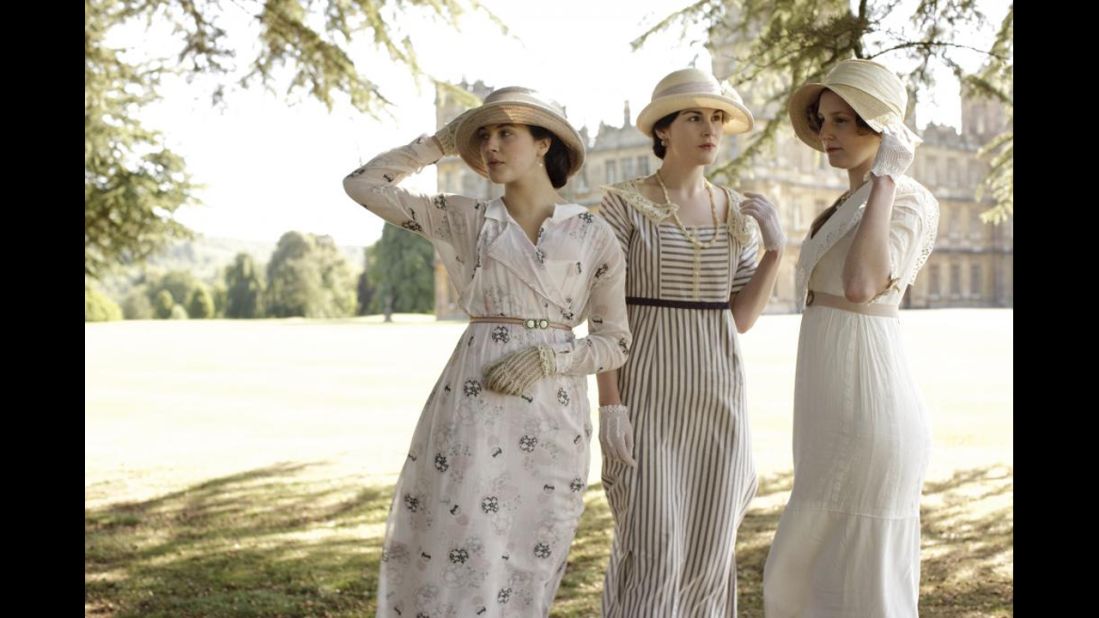In this image, there are three young women dressed in early 1900s-style attire, standing side by side in a grassy outdoor area. The photograph, which appears to be quite old and of moderate quality, captures them against the backdrop of a large, historic, castle-like building with rows of trees to its left. The sky above is cloudy, and the sunlight illuminates the grass around them.

The woman on the right is dressed in an all-white, long dress paired with white gloves and a beige belt. She wears a white hat and has her left hand touching the brim, possibly to keep it from being blown away by the wind. The central figure is attired in a white dress with black stripes and a thin black belt. She accessorizes with a pearl necklace and short white gloves, with her right hand resting at her waist and her left hand touching her shoulder. The woman on the left wears a white dress with blue designs and long sleeves. Similarly, she is holding her hat with her right hand as if to steady it against the wind. Each woman is looking in a different direction, adding to the dynamic feel of the scene.

Behind them lies a vast green lawn, with some bushes to the left and a hint of treetops in the upper left corner of the image. The overall scene evokes a sense of historical recreation or a homage to a bygone era.